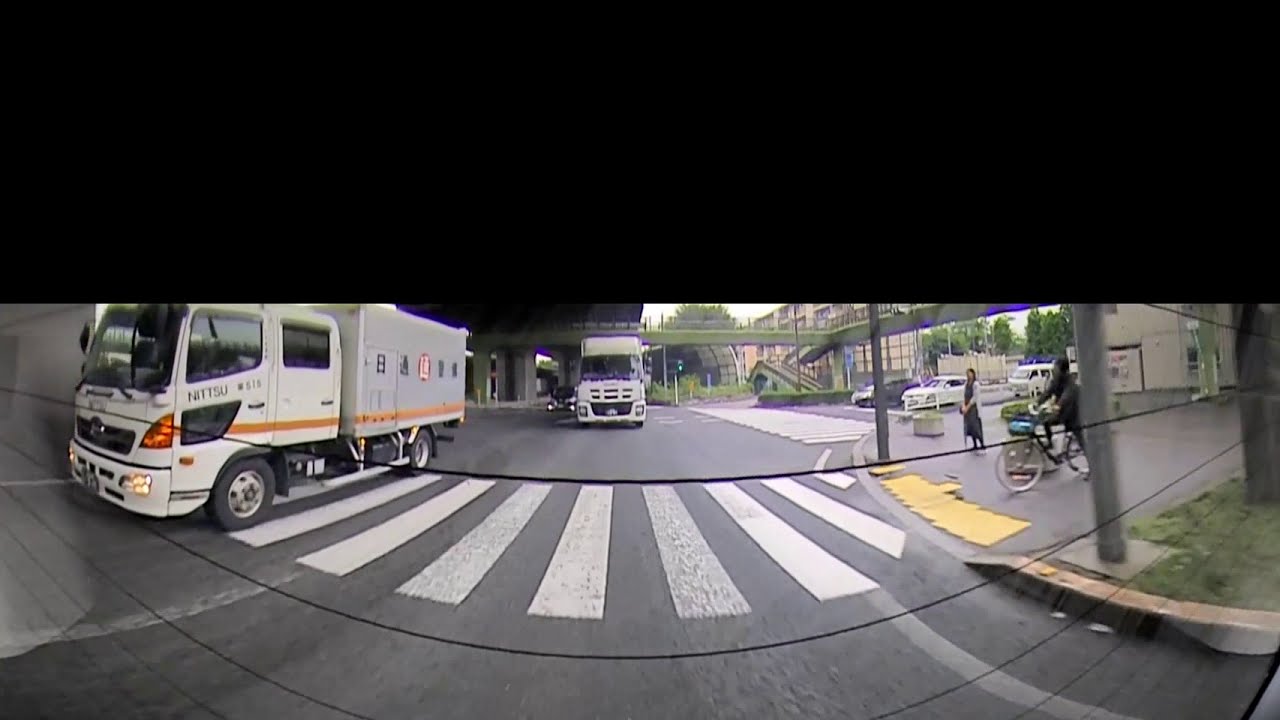In the foreground of the image, two large white trucks with long enclosed beds dominate the scene, positioned on a wide, grey concrete driveway with white stripes marking the pavement. One truck is situated to the left, poised near the grey concrete walls of a business with black engine lights on, while the other stands further back in the middle of the image. Behind the centrally located truck, a dark-colored car is visible. The driveway, beneath an awning supported by grey pillars, extends from the mid-point downwards, as a wide black stripe across the top of the image obscures the upper section. 

On the sidewalk adjacent to the driveway, a person clad in black rides a bicycle, passing by a lady who is standing nearby. A prominent pedestrian crossing cuts through the bottom of the scene where people are waiting to cross. In the background, a green-colored bridge connects to another structure, suggesting the trucks and cars are positioned near an overpass. The setting appears to be daytime in a relatively quiet city street, giving off the impression of a business area with light traffic.